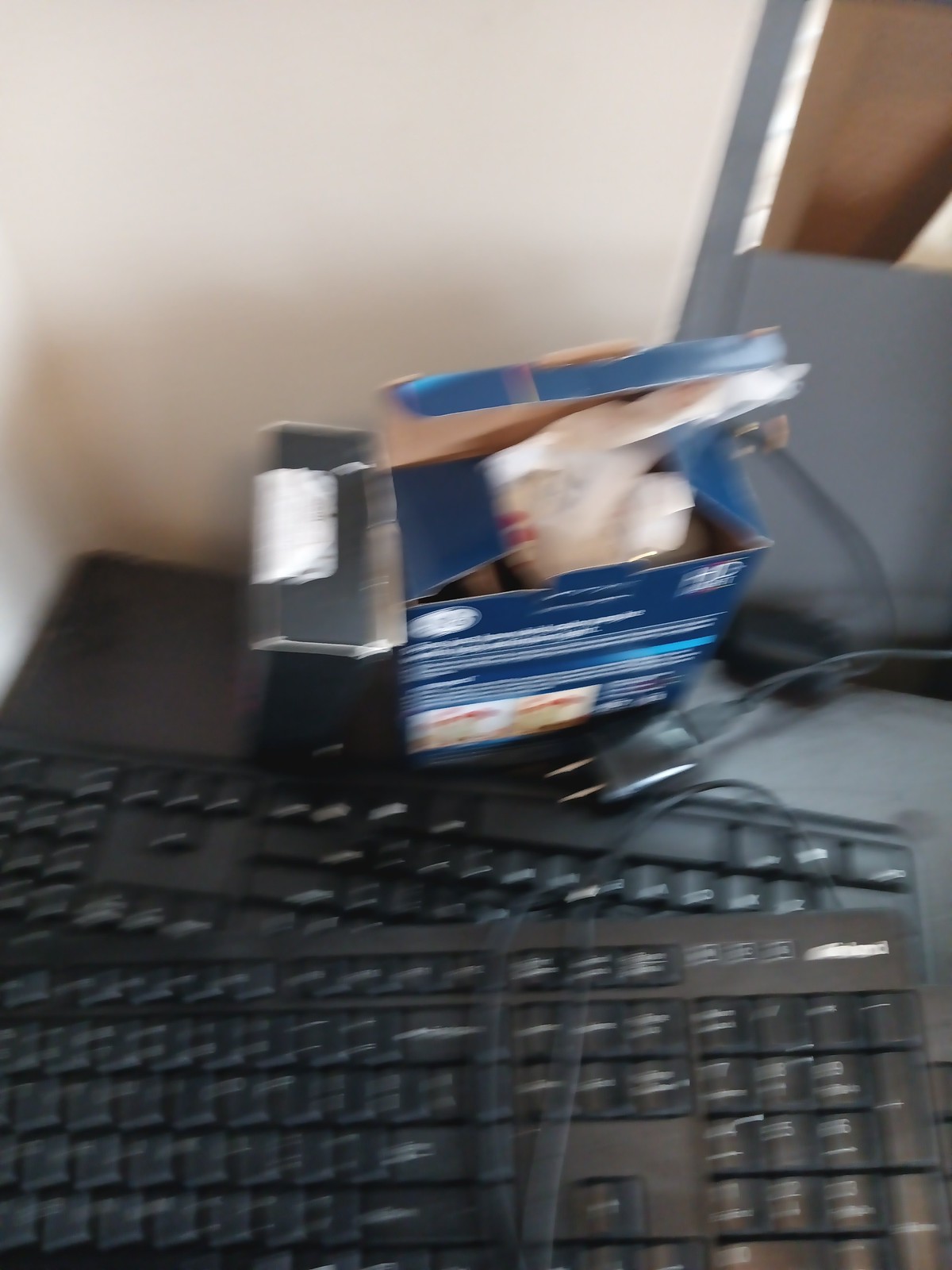On the beige-walled desk, two opened boxes are positioned side by side; one is blue with a visible white bag inside, and the other is black. In front of the boxes, two basic keyboards with numerical pads on the right-hand side are stacked on top of each other, their cords neatly wrapped around them as if prepared for storage. A charger, possibly for a phone, can also be seen in the background. The image is blurry, making the scene appear somewhat indistinct.